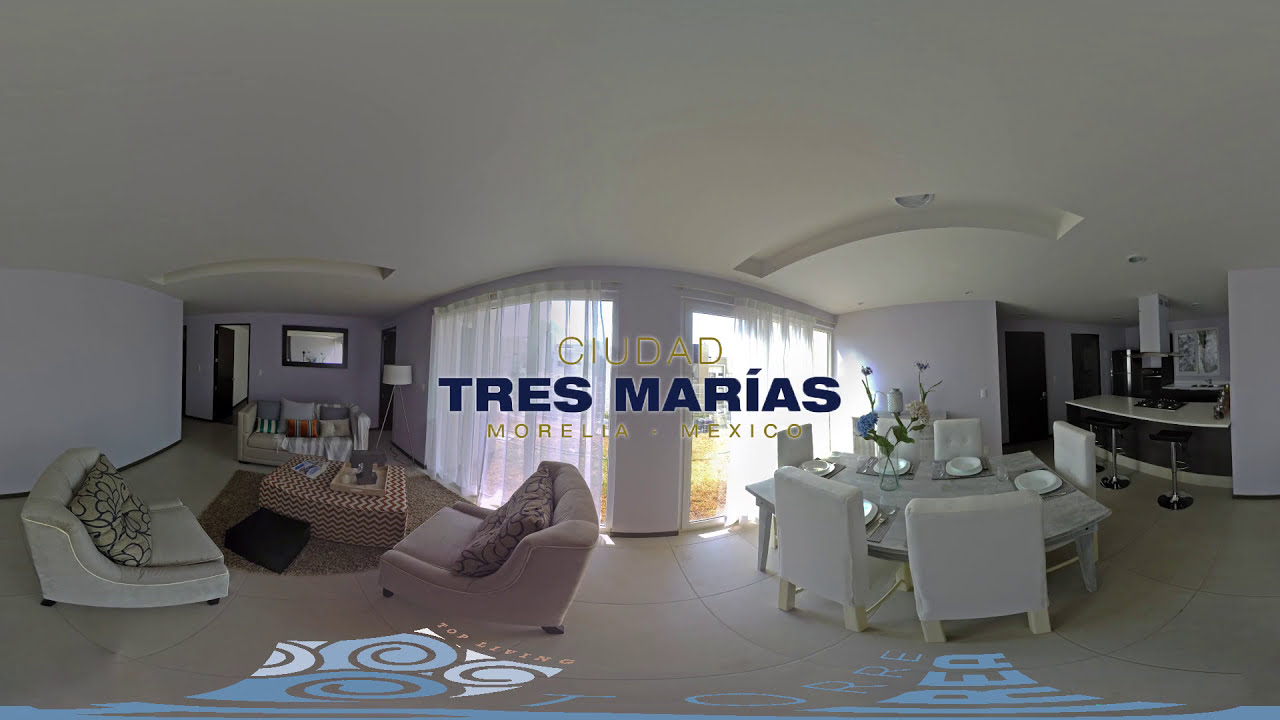This panoramic image showcases a spacious, elegantly designed room with distinct yet interconnected areas: a seating area, a dining area, a living room, and a bar/kitchen area. The entire room is predominantly white, featuring white walls, a smooth white tile floor, and a pristine white ceiling with recessed lighting arranged in an arched strip design. The floor-to-ceiling windows draped with sheer white curtains dominate the central view, curving slightly towards the front. 

The seating area to the left contains a loveseat and a pair of sitting chairs, one in beige and the others in white, arranged around a coffee table on a rug with a floor cushion nearby. Behind the loveseat, an open door and a mirror can be seen, enhancing the room's sense of space.

The dining area features a white table accompanied by six white chairs. Adjacent to it, a small pillar stands between the dining area and the sofa area, reinforcing the room's open-plan layout.

On the right side of the room, the bar/kitchen area presents a white countertop with three black bar stools. The black counter and a couple of black doors in the background add contrast to the predominantly white space. Above the central window area, a sign reads "CIUDAD Tresmarias" in yellow and bold blue letters, with "Morela, Mexico" in smaller yellow letters below.

Accentuating the serene and modern ambiance, soft violet hues subtly contrast on the walls, creating a balanced interplay of colors in this refined living space.